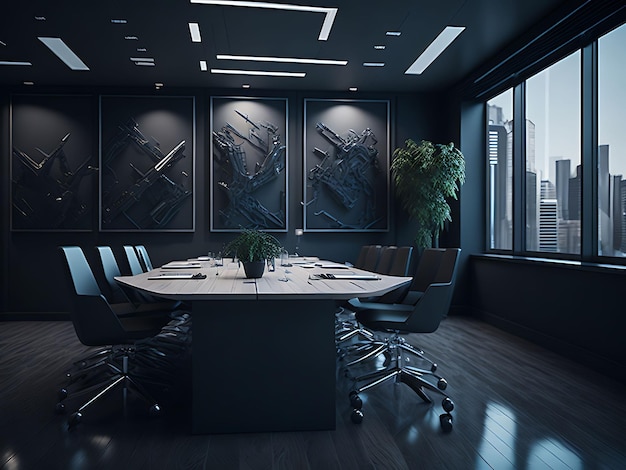The photograph captures a sophisticated, modern conference room situated on one of the higher floors of a skyscraper, as evidenced by the view of the tops of other skyscrapers through the long window stretching along one side of the room. The room features a large, light wooden table that stands out against the predominantly dark decor, which includes dark wood floors and black-painted walls. Eight black, wheeled office chairs are neatly arranged around the table, four on each side, with no chairs at either end. Each seat is equipped with what appears to be a clipboard or possibly a tablet, and there might also be glasses placed on the table. A small green plant serves as the central piece on the table, adding a touch of color. In the far corner near the window, a larger potted plant is positioned, contrasting with the sleek, modern elements of the room. The black walls are adorned with abstract metal sculptures, described by some as resembling weapons, giving an edgy yet contemporary feel. The ceiling features recessed, rectangular lighting that complements the room's stylish and dark aesthetic.